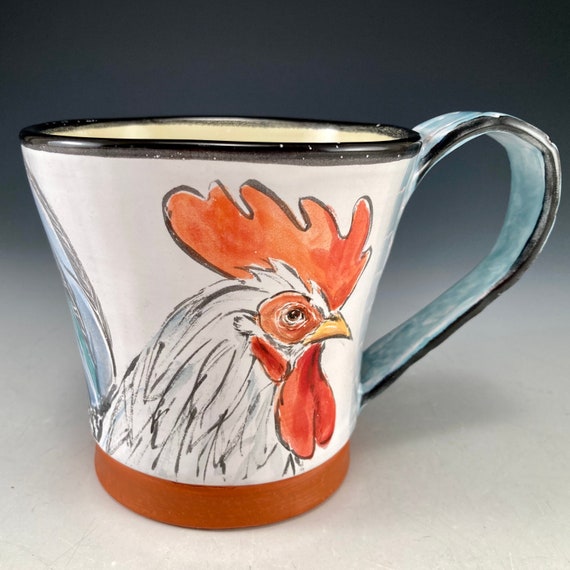The image showcases a meticulously decorated ceramic cup, prominently occupying the entire frame. Adorned with a charming chicken head motif, the cup features a vibrant palette of colors, including shades of orange, white, black, light blue, dark blue, and brown. The cup rests on what seems to be a floor, devoid of any accompanying text. Captured by a photographer without the aid of AI technology, the photograph purely highlights the artistic intricacies and vibrant hues of the rooster-themed cup.